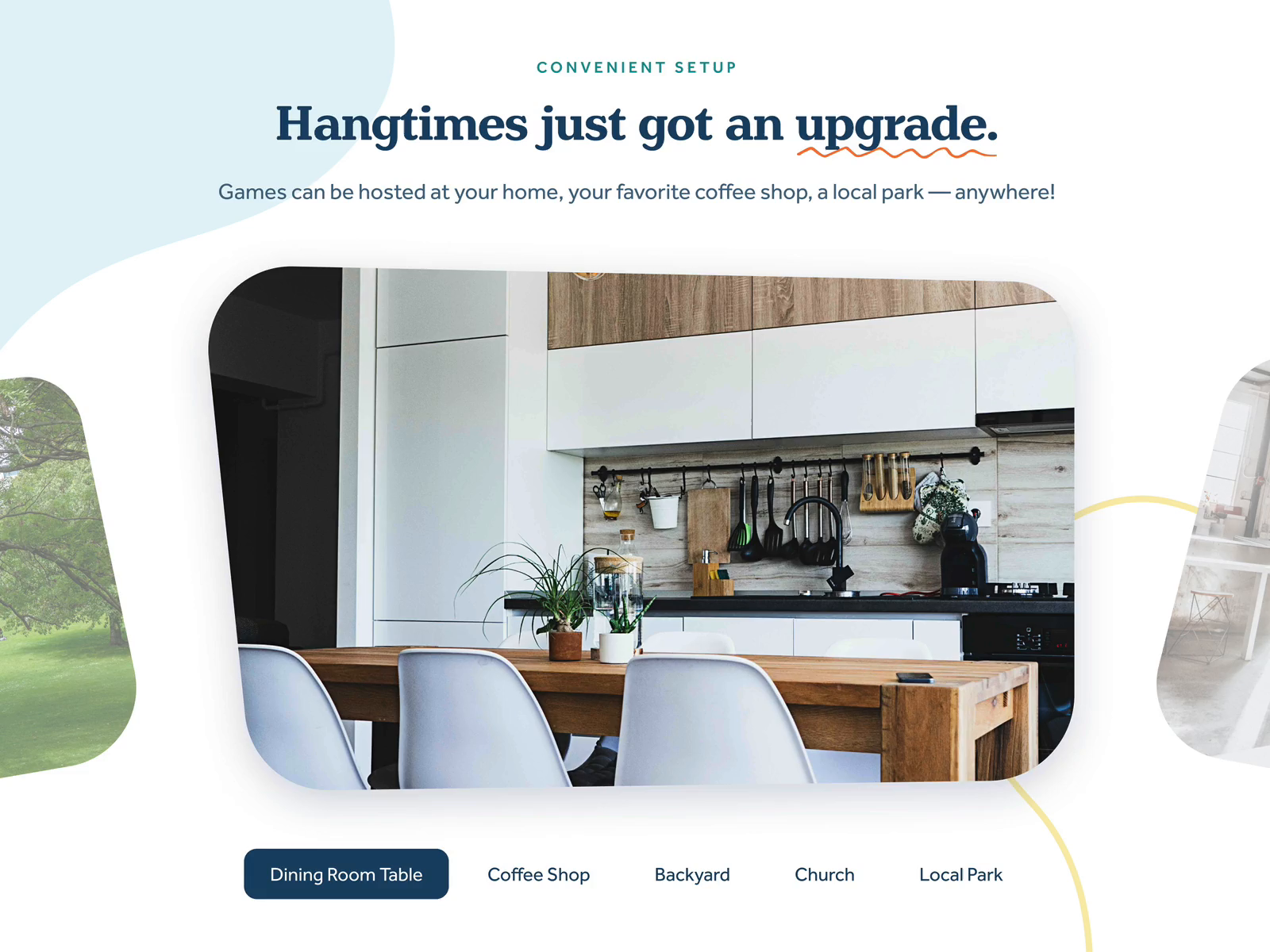This landscape-oriented advertisement is set against a white background, featuring a prominent central image and grayed-out, out-of-focus images on the sides. The main image, slightly longer than it is tall, boasts a blue spot in the top corner and a header. At the top center, in varying fonts and colors, it reads: "Convenience setup" followed by "Hang times just got an upgrade" in large, dark blue font with a yellow squiggly line underneath the word "upgrade," mimicking a Microsoft Word error underline. Beneath this, a subheadline indicates that, "Games can be hosted at your home, your favorite coffee shop, and a local park, anywhere."

Positioned below this text, a uniquely shaped image begins as a rectangle with rounded edges before the upper left corner extends out into a vertical line, resembling a trapezoid. This image depicts a cozy kitchen featuring a wooden table with three white chairs against a white wall. The kitchen setting is complete with a stove, countertops, and various kitchen utensils such as pans, pots, and spatulas hanging on a black wall with a drying rack.

Towards the bottom of the advertisement, there is a list of venue options for hosting. One option, "Blue table," stands out in a rectangular blue box with white font, while additional options—"Coffee shop," "Backyard," "Church," and "Local park"—are displayed in blue font against a white background.